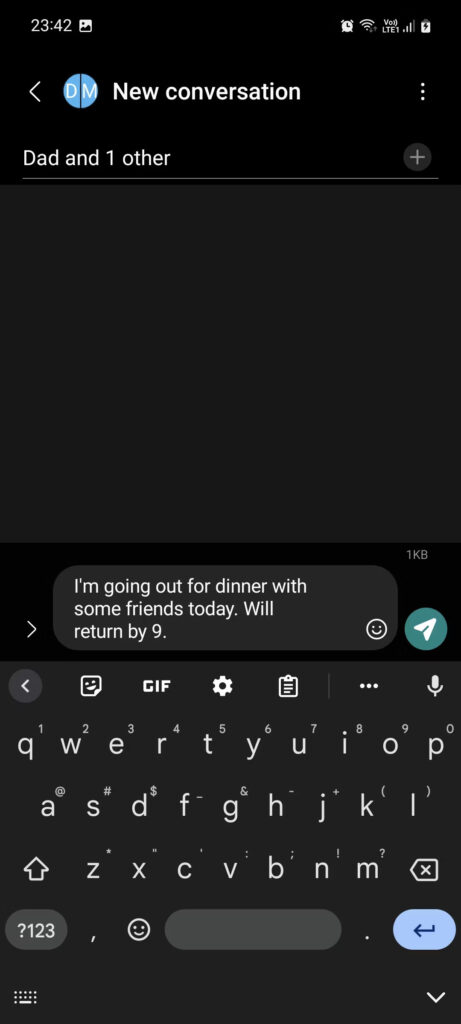In the image, there is a screenshot of a smartphone displaying a messaging app. The screen is titled "New Conversation," with icons representing the participants: a blue circle with a "D," likely signifying "Dad," and a green circle with an "M," possibly representing the sender. The time at the top of the screen is 23:42. On the right side of the header, there are icons indicating the phone’s status, including a clock, Wi-Fi strength, signal bars, and a partially charged battery.

Below the header, there is a blank conversation space, indicating no prior messages between the participants. At the very bottom of the screen, a message has been composed: "I'm going out for dinner with some friends today, will return by 9." Next to the text input area, there is an emoji icon that allows the sender to add an emoji to the message. There is also a send button resembling a paper airplane inside a green circle, ready for the message to be sent. The layout suggests that additional text can be typed if needed.